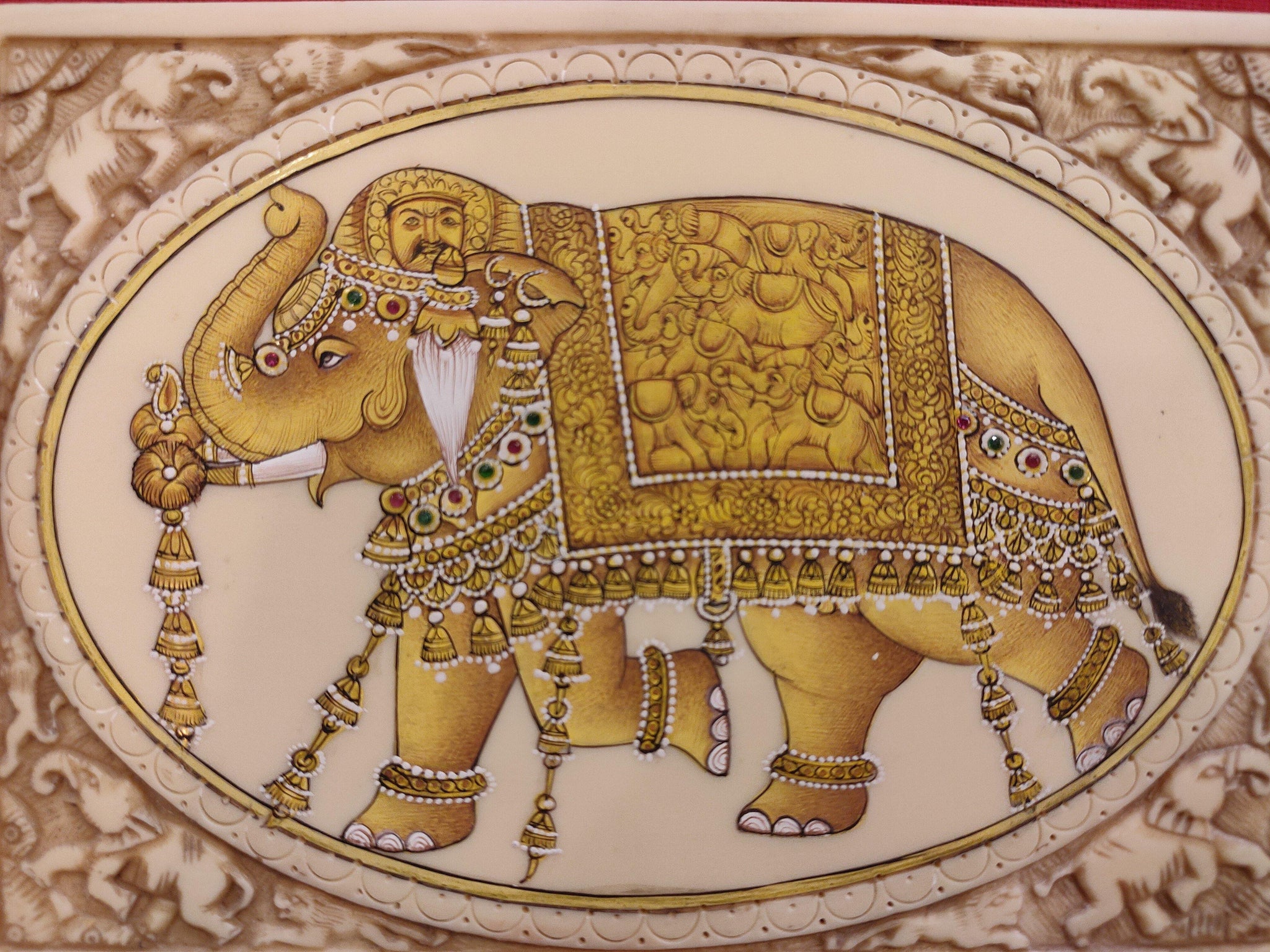The image features a golden elephant adorned with an opulent, highly detailed array of decorations and jewelry typical of Indian craftsmanship. It stands within a cream-colored circular frame with a gold ring accent. The elephant is richly adorned with a yellow, tapestry-style rug draped over its back, fringed with yellow bell-like ornaments. Red and green jewel-like embellishments are meticulously arranged on the straps that secure the tapestry across its chest and rear.

The elephant's ears are pierced, showcasing yellow fringe tassels. A striking element is a man's face, resembling traditional Asian artistic depictions, complete with a wispy black mustache and black eyebrows, positioned on top of the elephant's head. From this face, a white, paintbrush-like tassel hangs down.

The elephant’s tusks are decorated with circular, flower-like ornaments adorned with yellow fringe bells. Each foot is encircled by a yellow bracelet studded with white pearls. The entire ensemble rests on an ivory dish embellished with half-circle patterns and is bordered by a rectangular carved ivory frame featuring a procession of elephants and lions.

The golden elephant itself is visually elevated by additional details—a sash or blanket decorated with patterns of more elephants, and its trunk raised towards the air. The overall scene is intricately engraved, creating a mesmerizing and ornate depiction of this majestic, jewel-bedecked elephant against the luxurious backdrop.